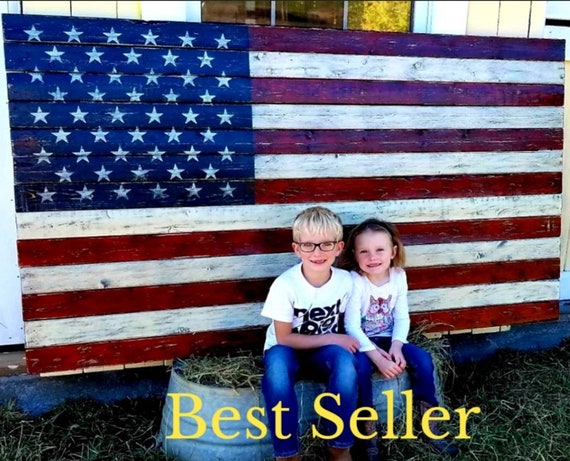In this realistic horizontally-oriented photograph, two young children, a boy and a girl, are sitting outside on upside-down aluminum or tin buckets filled with hay. They are positioned in front of a large American flag made of wooden planks, painted in the traditional red, white, and blue colors with white stars on a blue field. The flag leans against a building constructed of vertically-oriented white wooden planks, featuring a prominent window that adds depth to the background. The boy, who appears to be around five years old, has blonde hair and wears glasses, a short sleeve white t-shirt with black lettering, and blue jeans. The girl, approximately four years old, has brown hair and is dressed similarly in blue jeans and a long sleeve white shirt adorned with an owl design. Both children are surrounded by scattered hay on the ground. At the bottom of the image, the word "bestseller" is displayed in bold yellow font, suggesting perhaps a thematic or promotional element to the scene.